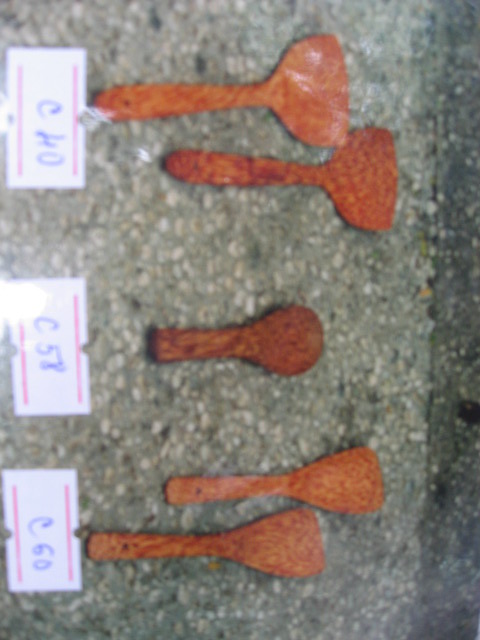In this slightly blurry photograph taken from a sideways angle, five kitchen utensils, resembling spatulas and spoons, are meticulously arranged on a gray concrete surface. They exhibit varying shades of orange, red, and brown. The arrangement includes two larger spatulas at the top, followed by a smaller spoon-like utensil in the middle, and two slimmer spatulas at the bottom. Each utensil rests on a white card, bordered with red lines, and the cards bear labels in blue lettering. The labels are as follows: the top pair is marked "C40," the middle spoon is labeled "C58," and the bottom pair is denoted "C60." This detailed layout emphasizes both the unique design of each utensil and the systematic method of labeling them.